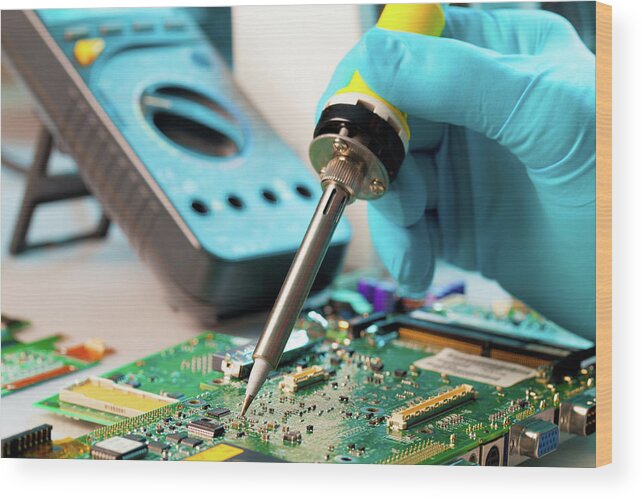The photograph captures a detailed scene of a computer motherboard, occupying almost the entire lower half of the image. A hand, donned in a blue rubber glove likely to prevent electrical shock, is prominently positioned over the motherboard. This hand holds a yellow-handled tool with a metal, pencil-like point, indicative of a soldering iron. The tool, attached to the handle with screws and a black band near its top, is directed towards the motherboard, suggesting a soldering operation. The left portion of the image features a large device resembling a phone case, with a turquoise face, a central dial, and four black dots underneath – possibly indicating areas that light up. This instrument, likely used to test the motherboard’s functionality, has a metal border and stands out amidst the blurred background, enhancing the focus on the detailed scene in the foreground. Vibrant yellows, greens, and blacks prevalent in the scene further accentuate the various components and intricate details of the motherboard.